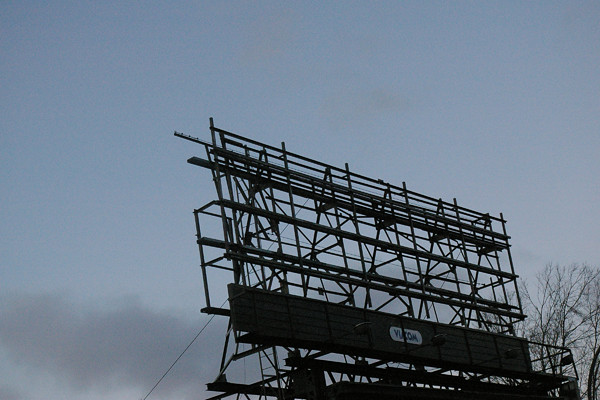This photograph captures the stark frame of an empty billboard, its metallic bars crisscrossing in a structural lattice. The billboard frame is painted black, and though there's a white logo on the front, it is indecipherable. In front of the frame, a small platform appears, complete with steps leading up to it, suggesting a space accessible for maintenance or installation. Bare treetops form a sparse backdrop, their branches stripped of foliage, contrasting with the low-hanging gray clouds that cast a somber tone over the scene. Above, the sky transitions to a clearer, albeit grayish-blue hue, offering a muted yet tranquil canopy over this desolate urban structure.